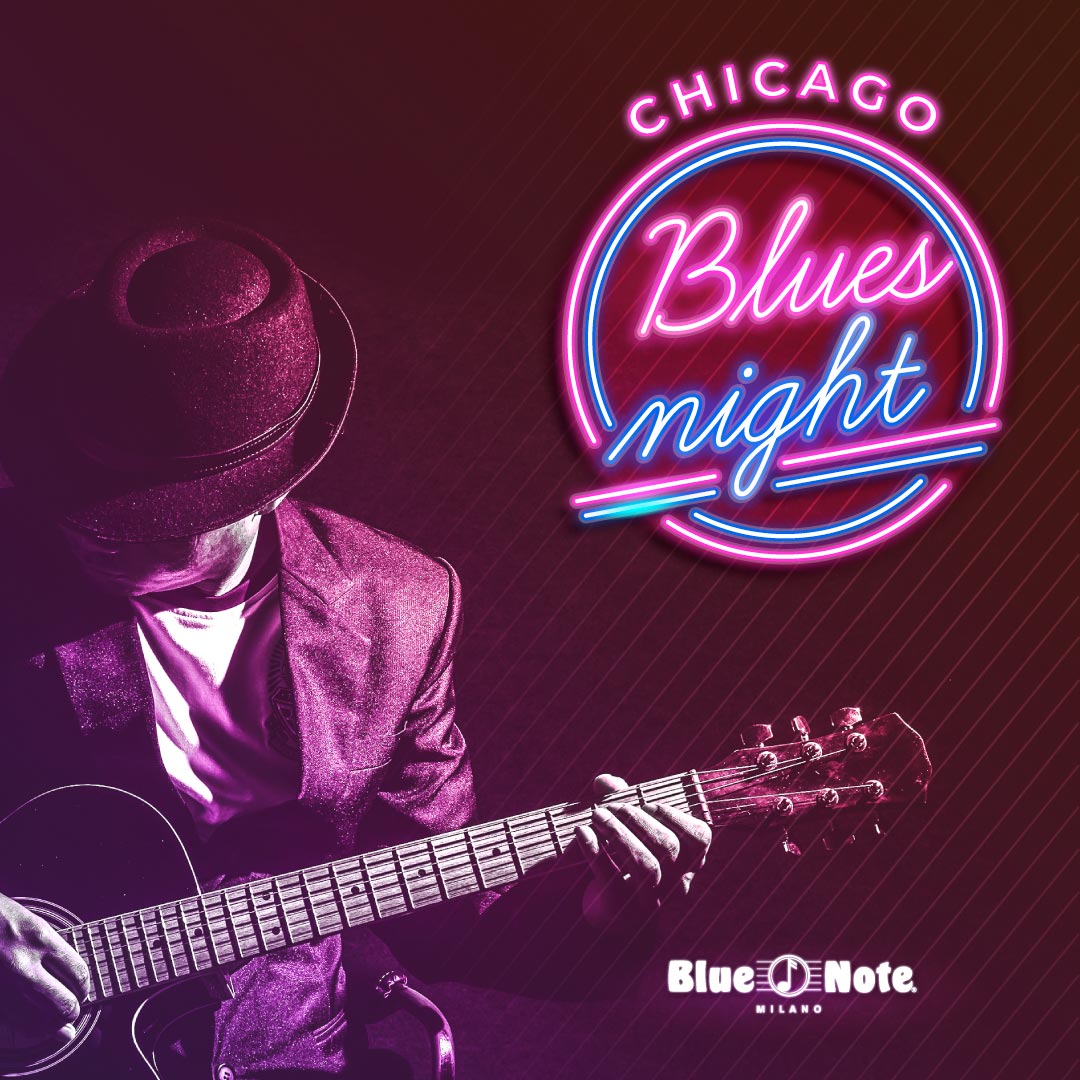This advertisement showcases "Chicago Blues Night" with a distinct neon-themed design. The vibrant logo is positioned in the upper right corner, featuring "Chicago" in pink neon above a circular emblem, within which "Blues Night" is displayed using pink and blue neon lights, double underlined with matching neon lines that subtly integrate with the logo's elements. The entire image is bathed in a purple hue, creating a visually captivating backdrop. To the left side, a man is depicted playing an acoustic guitar; his face concealed by a brimmed hat as he looks downward. He wears a black suit jacket over a light-colored shirt, illuminated in the neon glow, amplifying the mysterious atmosphere. In the lower right corner, there's a "Blue Note" logo, styled in white text with a musical note icon, followed by "Milano," suggesting the business behind the event. The background also features faint white diagonal lines concentrated in the bottom right quadrant, enhancing the overall dynamic design of the poster.